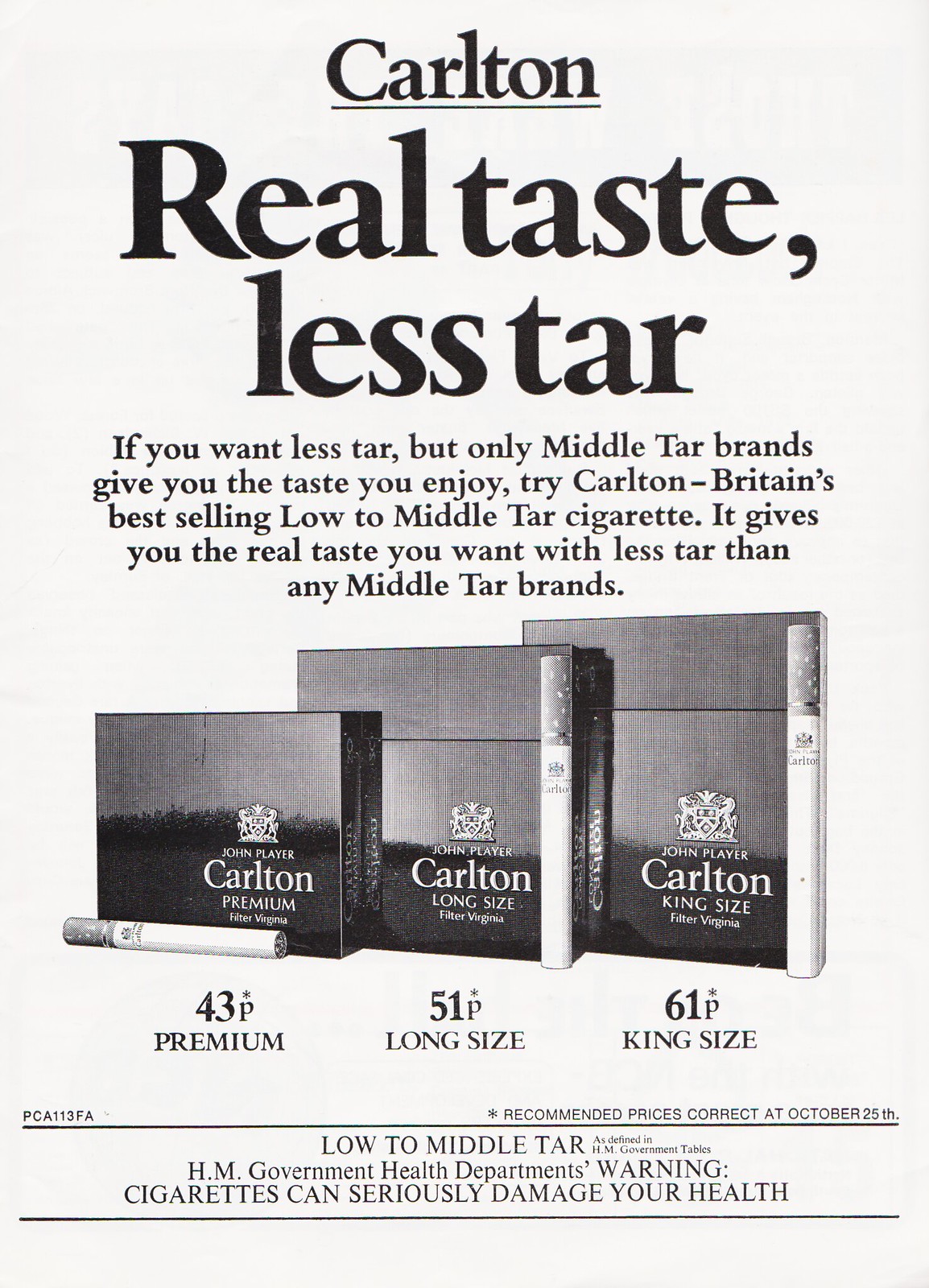This black-and-white vintage cigarette advertisement, resembling a magazine print, promotes Carlton cigarettes. At the top, large black text reads "Carlton," followed by the headline "Real Taste, Less Tar." Below the headline, a detailed paragraph describes Carlton as Britain's best-selling low-to-middle-tar cigarette, emphasizing its claim to provide real taste with less tar than other middle-tar brands.

The central image features three packs of Carlton cigarettes, each showcasing different sizes: 43 premium, 51 long size, and 61 king size. The smallest pack, priced at 43p, lies horizontally on the left, while the progressively larger 51p and 61p packs stand vertically beside it. The cigarettes themselves are gray in color, matching the grayscale theme of the ad.

At the bottom of the advertisement, a government health department warning in small black text alerts consumers that "Cigarettes can seriously damage your health" and notes that the product has low to middle tar content. This combination of photography and graphic design typography gives the ad a classic, nostalgic feel, capturing the essence of vintage print publications.